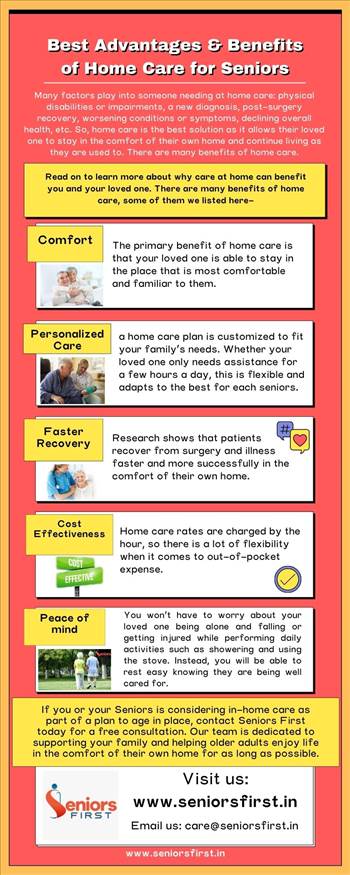The image features a pamphlet titled "Best Advantages and Benefits of Home Care for Seniors," framed by a gold border. This advertisement from Seniors First uses a combination of red, yellow, and white colors. Under the main heading, the text is too small to discern clearly, but it mentions several key factors necessitating at-home care, such as physical disabilities, new medical diagnoses, post-surgery recovery, worsening conditions, and declining overall health. The pamphlet highlights five main benefits of home care: comfort, personalized care, faster recovery, cost-effectiveness, and peace of mind. A yellow caption encourages readers to learn more about these advantages. Additionally, contact details are provided at the bottom, including a website (www.seniorsfirst.in) and an email address, emphasizing the informative nature of the pamphlet that aims to advocate for in-home senior care.